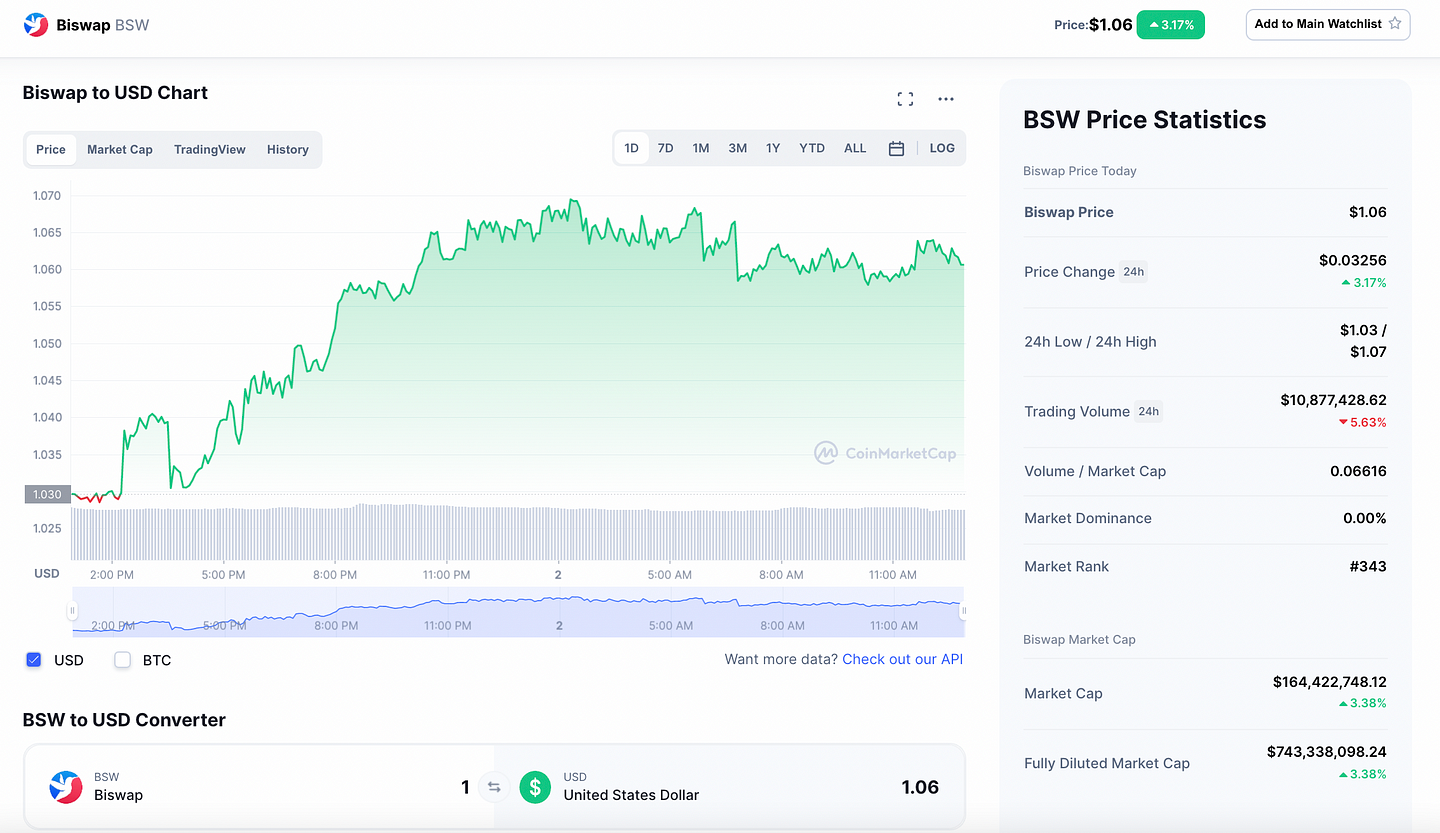The image depicts a detailed page of BySwap (BSW) cryptocurrency statistics. At the top, "BySwap BSW" is prominently displayed alongside an icon featuring blue, white, and red colors, set against a white background with predominantly black text. The current price of BySwap is shown as $1.06, highlighted by a green icon indicating that the price has increased by 3.17%.

An option to add BySwap to the main watchlist is available, marked by a star icon. The section titled "BSW Price Statistics" provides comprehensive data, including the following:

- **BySwap Price:** $1.06
- **Price Change in the Last 24 Hours:** Up 3.17%
- **24-Hour Low:** $1.03
- **24-Hour High:** $1.07
- **Trading Volume (24 Hours):** Down 5.63%
- **Market Cap:** 0.06616
- **Market Dominance:** 0%
- **Market Rank:** 343

At the bottom of the page, additional details are provided, such as a BSW to USD converter indicating that one BySwap is equivalent to $1.06. 

The page also features a large comparative graph charting the price of BySwap against the US Dollar (USD), with an option to compare it to Bitcoin. The graph is predominantly green, showcasing a gradual upward trend in BySwap’s price.